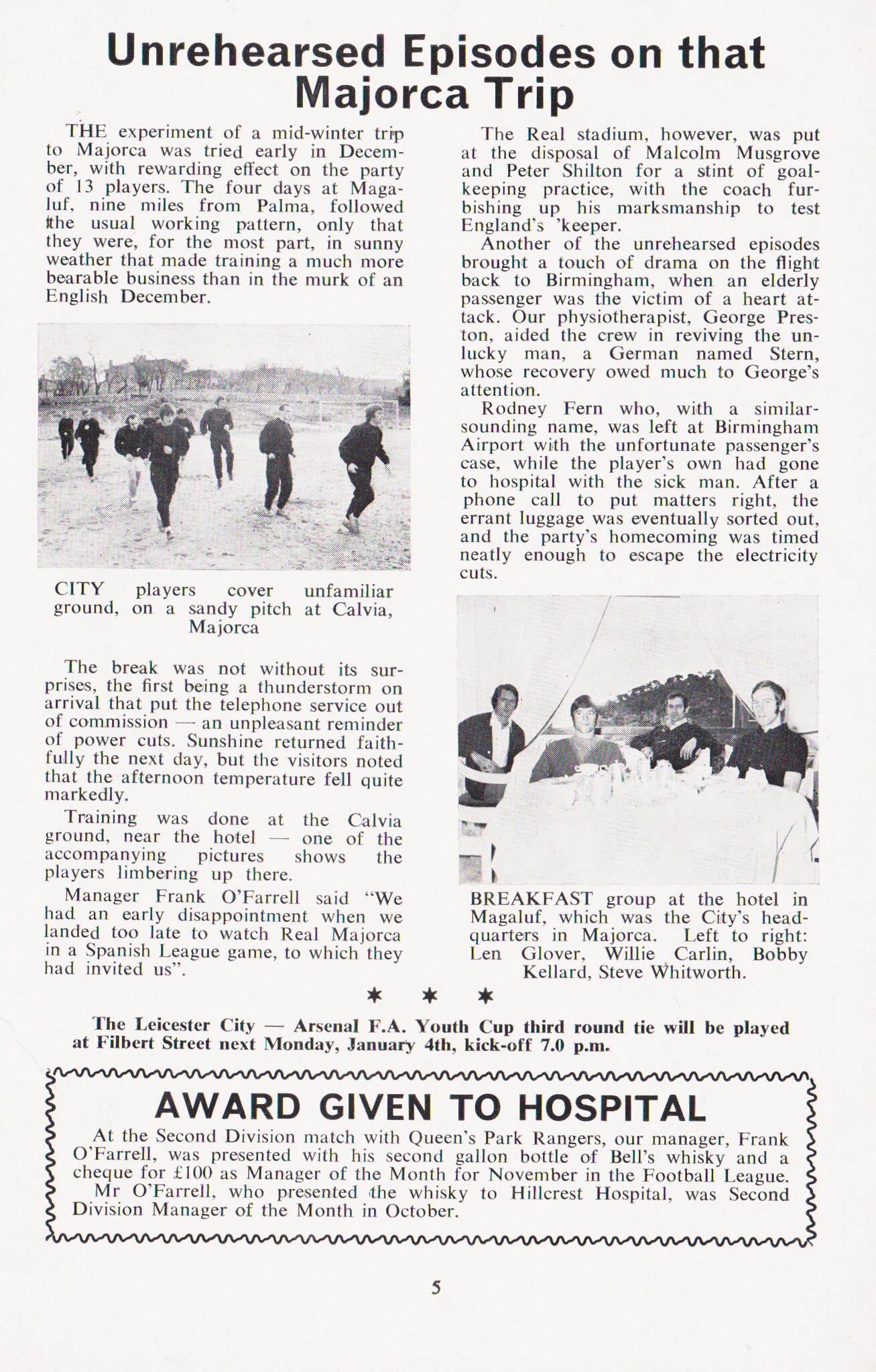This black and white clipping, likely from a newspaper or magazine, features an article titled "Unrehearsed Episodes on That Mallorca Trip," chronicling the events of an English football team's visit to Mallorca. The page, about 5 inches wide and 8 inches long, is arranged in two columns of text. The left column highlights the team training on a sandy pitch in Calvia, near their hotel, with a photograph of players in sweatsuits running in the field. The right column delves into various activities during their stay, including a dramatic flight back to Birmingham where a physiotherapist attended to an elderly passenger suffering a heart attack.

The first column details the initial disappointment of missing a Spanish league game and the team's training sessions at the Calvia Ground. A quote from Manager Frank O'Turillo recalls, "We had an early disappointment when something landed too late to watch something Mallorca in a Spanish league game to which they had invited us." Completing this column is a description of the city players covering unfamiliar ground on a sandy pitch, with a scenic view implied due to Mallorca being an island off the coast of Spain.

The second column features the breakfast group at the team's hotel in Magaluf, Mallorca, captioned with the players' names: Len Glover, Willie Carlin, Bobby Kellard, and Steve Whitworth. The column continues with an account of the flight back to Birmingham, where team members assisted a heart attack victim and ensured their party's homecoming was unaffected by electricity cuts. Below the text, three stars indicate an additional note spans both columns, highlighting an upcoming Leicester City Arsenal FA Youth Cup match.

At the bottom of the page, beneath the text, is a small box with the typewritten note, "Award Given to Hospital," which mentions Hillcrest Hospital's accolade from October. The overall presentation and content suggest it is a historical piece from a period with typewriter-era formatting.